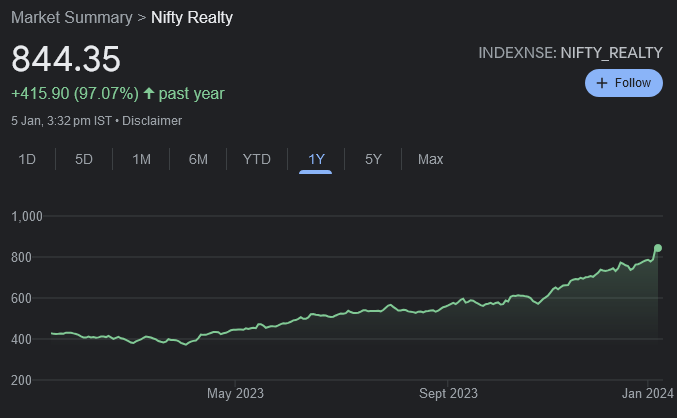In this screenshot, we see a detailed market summary graph with a predominantly black background. The main text, displayed in white, shows a value of $844.35, indicating a positive change with +$415.90 (97.07%), accompanied by an upward-pointing arrow. The time frame referred to is "past year," specifically captured on January 5th at 3:32 PM. A light gray disclaimer is also visible.

The graph features various time selection options: 1D, 5D, 1M, 6M, YTD, 1Y, 5Y, and MAX. The x-axis is marked with key dates, including May 23rd and January 24th, while the y-axis is labeled with numerical values: 200, 400, 600, 800, and 1000. The graph itself showcases a jagged neon green line that begins near the 400 mark and gradually ascends throughout the year, ultimately surpassing the 800 mark by January.